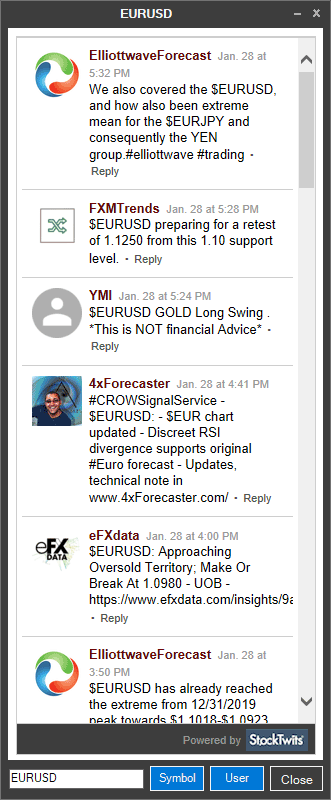This image appears to be a screenshot taken from a mobile device, possibly from a financial or trading application. It is formatted in a vertical layout, divided into six distinct sections, each separated by thin gray horizontal lines. At the very top, in the center, the text "EURUSD" is prominently displayed in a white font, contrasting against a dull black outline that encircles the entire image. Additionally, there is a thin gray vertical line running from the top to the bottom of the image, further segmenting the content.

Within the black frame, a vertical scroll bar can be seen on the right side, suggesting that there is more content available for scrolling. The topmost section is labeled "Elliott Wave Forecast," timestamped with "January 28th at 5:30 p.m." directly below it, organization titles follow: "FXM Trends," "YMI," "Forex Forecaster," and "EFX Data," each occupying its own respective section. The detailed labels and timestamps indicate that this image likely pertains to real-time financial data analysis or updates.